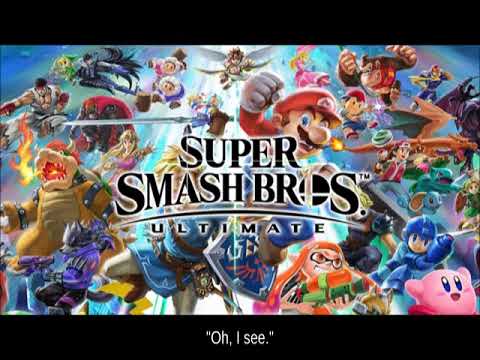The image is a vibrant, advertisement for the Nintendo game "Super Smash Bros. Ultimate." The background showcases an exhilarating array of popular Nintendo characters in a kaleidoscope of colors, including Mario, Bowser, Kirby, Donkey Kong, Zelda, Mega Man, Ryu from Street Fighter, Captain Falcon, Kid Icarus, Fox from Star Fox, and Link from Zelda. The central logo features "Super Smash Bros." with a superscripted trademark symbol (TM), underscored by a curved line, followed by the word "Ultimate" in striking black font. Notably, Mario is depicted with his fist outstretched, and Bowser is dramatically captured breathing fire. Positioned prominently in the center, Mario and Zelda stand out among the densely packed characters. Black letterbox bars border the top and bottom of the image, enhancing a cinematic feel. At the bottom, a caption in white letters and quotation marks reads "OIC," adding a unique touch to the dynamic scene.